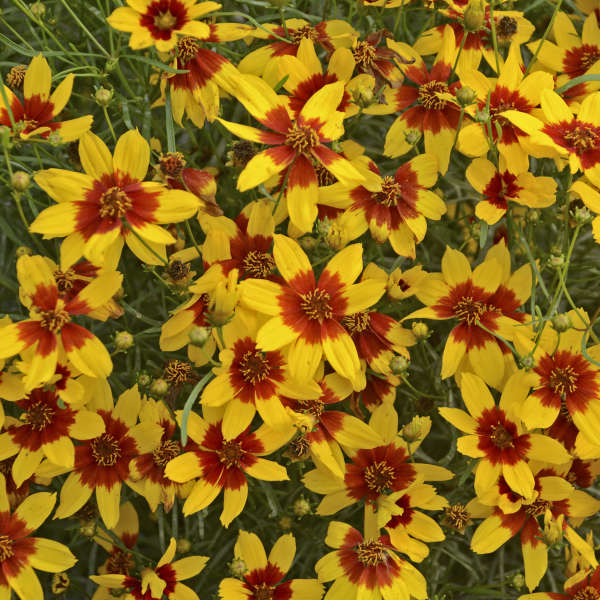The photograph is a stunning close-up view of a field of golden yellow flowers, captured in the natural daylight. Each flower is tightly bunched together with stems and thin grass-like leaves that create a lush green backdrop. The flowers, displaying seven to eight petals each, exhibit a radiant yellow hue on the outer edges that transitions to a vibrant sunburst of orange or red towards the middle. The very centers of the flowers are even darker orange or red, featuring yellow protrusions that seem to reach out and create a striking contrast. Additional unbloomed green buds are also scattered among the open flowers, hinting at the vitality of the entire field. The overall composition taken from a top-down perspective showcases the densely packed flowers, covering the entire frame and capturing the essence of nature in full bloom.